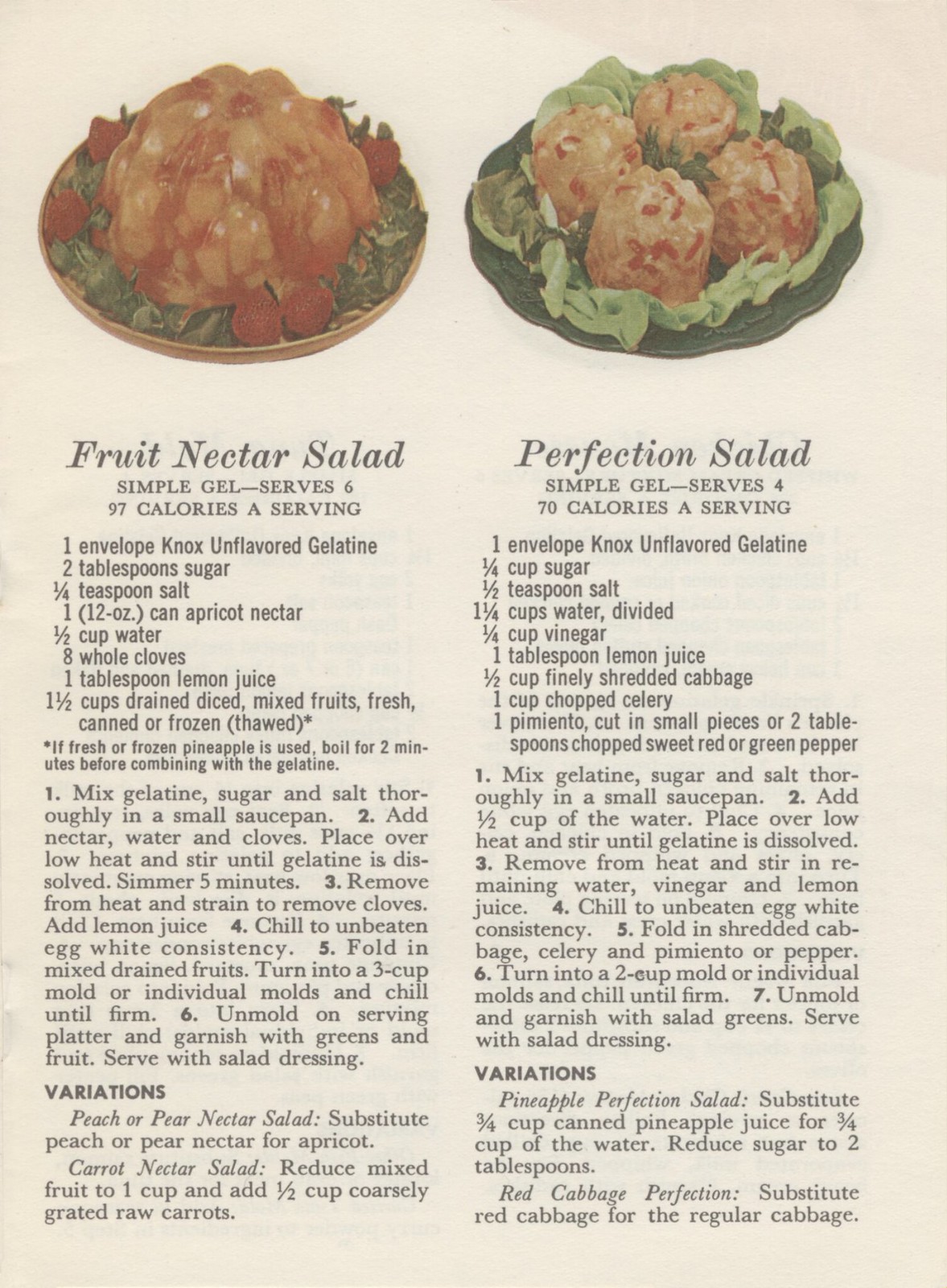This image is a photograph or print of a vintage magazine or newspaper page, likely from the late 1950s or early 1960s, showcasing two old-fashioned Jell-O salad recipes. The page is presented on a white background with two columns, each featuring a recipe both with detailed descriptions and their corresponding images at the top.

On the left, the recipe titled "Fruit Nectar Salad" includes a colorful image of a circular Jell-O mold, tinted yellow, embedded with fruit pieces and garnished with strawberries and green leaves, possibly lettuce or spinach. The recipe mentions that it serves a simple Jell-O dish containing 97 calories per serving.

On the right, the "Perfection Salad" recipe features four individual Jell-O servings that are also yellow with visible red pieces, each presented in a small mold atop lettuce leaves. This recipe states it serves a Jell-O dish with 70 calories per serving.

Below each image, the detailed list of ingredients and instructions provide additional directions for preparing the salads, with the left column dedicated to "Fruit Nectar Salad" and the right to "Perfection Salad." Additionally, there are variations and tips included at the bottom. The overall layout and aesthetic suggest it is an advertisement for Knox Unflavored Gelatin.